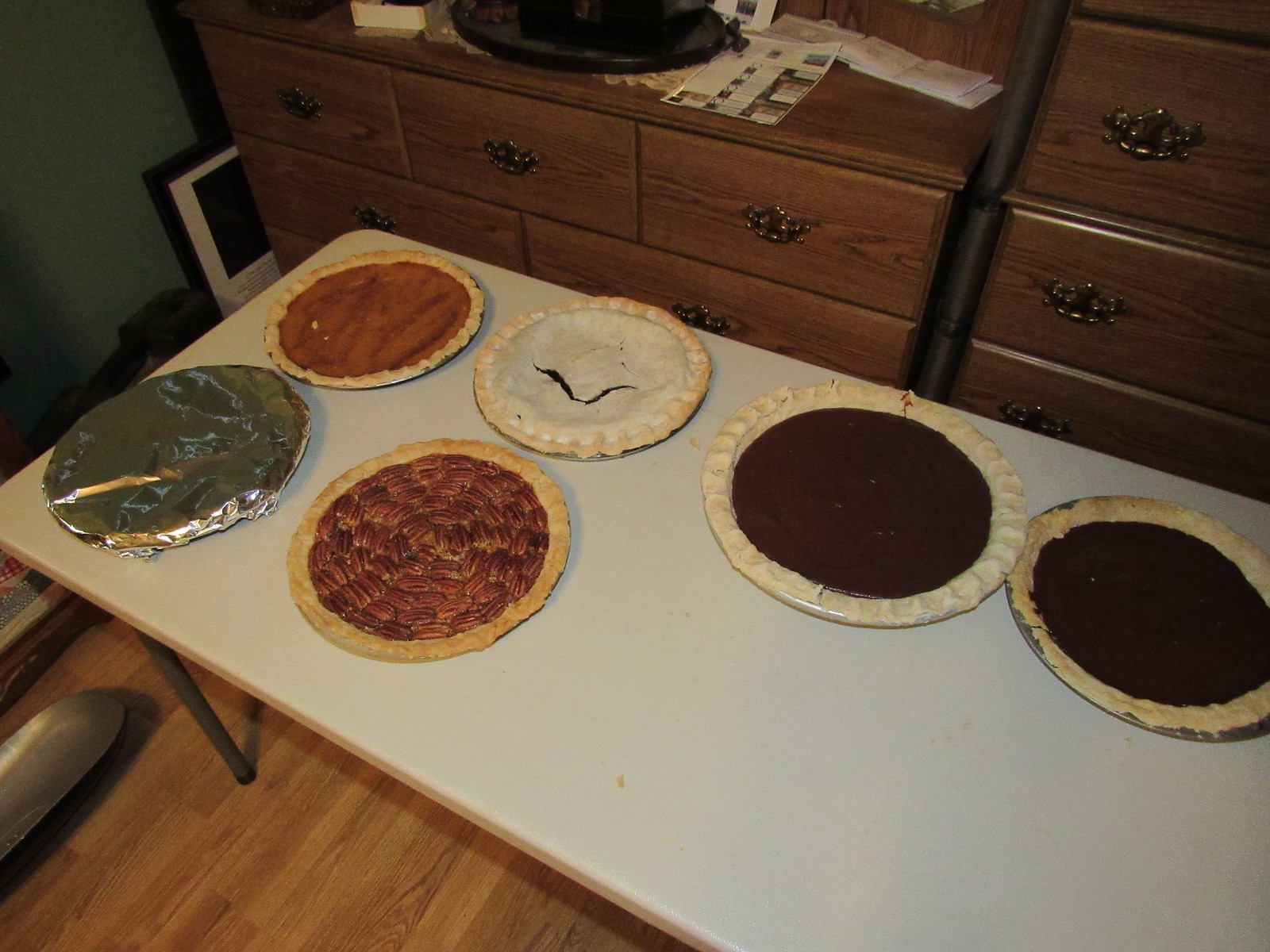This photograph, taken from above, provides a detailed look at a scene featuring six pies arranged on a white folding table with gray metal legs, set against a medium brown wood floor. To the left of the table, there are two oakwood dressers with brass-colored handles, one of which is partially cut off by the edge of the image. The room appears to have an olive green wall behind these dressers. The pies, arranged in two rows with four on top and two on the bottom, seem to be homemade and brought out for a special occasion, possibly a potluck dinner. Starting from the top left, there is a pumpkin pie followed by a fruit pie that might be blueberry, identifiable by a crack in its top crust. Next, there are two chocolate cream pies. On the bottom row, the left pie is covered in tinfoil, masking its identity, and the last pie is a pecan pie. The table's positioning suggests it has been brought out specifically for this event, as it is placed in close proximity to the dressers, which also have some stored materials behind them.